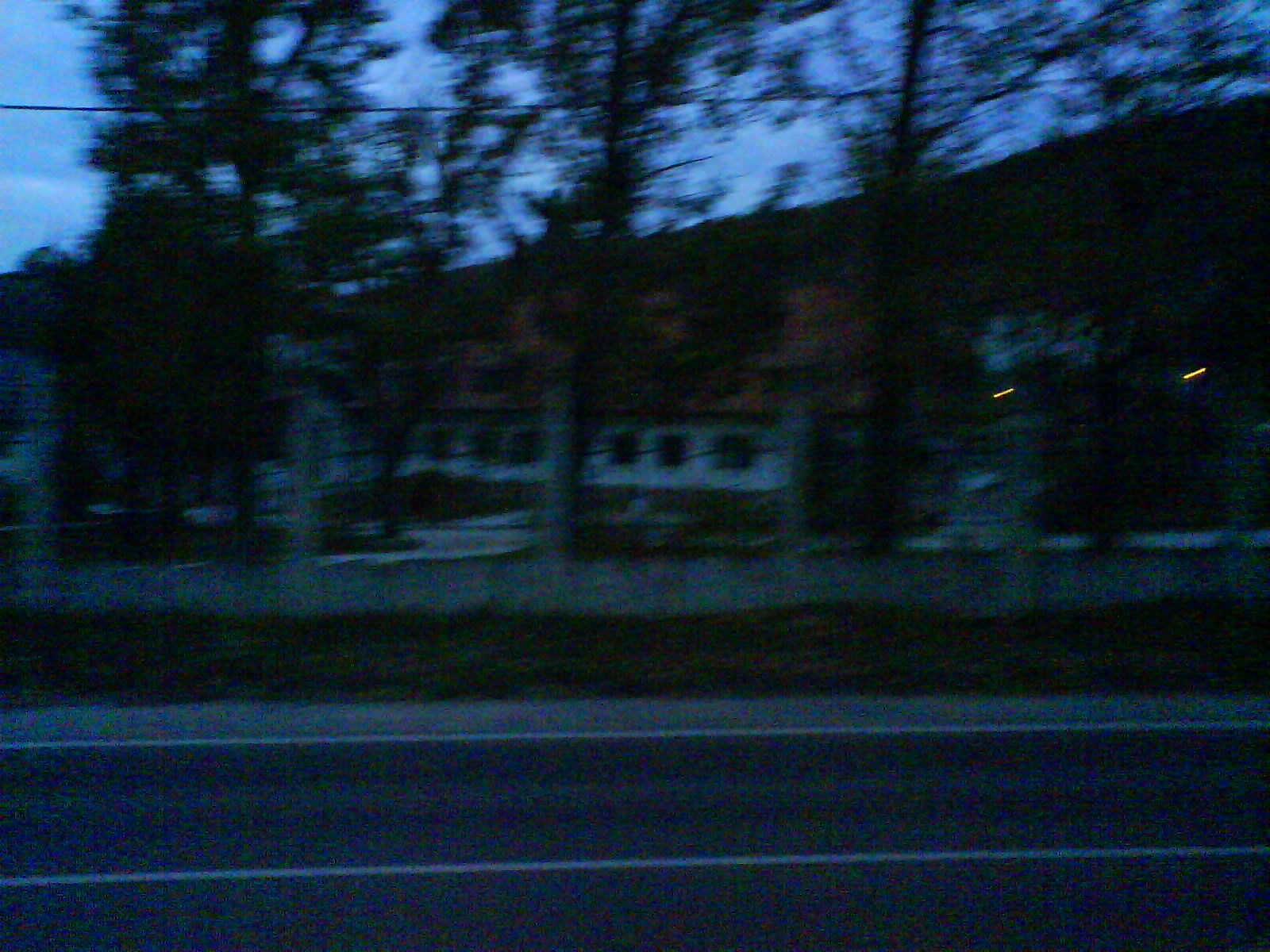The image is a blurry, low-quality, low-resolution square photograph capturing an outdoor scene. The sky, predominantly white and light blue, spans the upper portion of the image. Below the sky, a black road with a white line running horizontally from left to right is visible. Behind the road, there is a field of green grass stretching across the width of the image. Further into the background, at least four trees can be discerned, despite the overall fuzziness of the image.